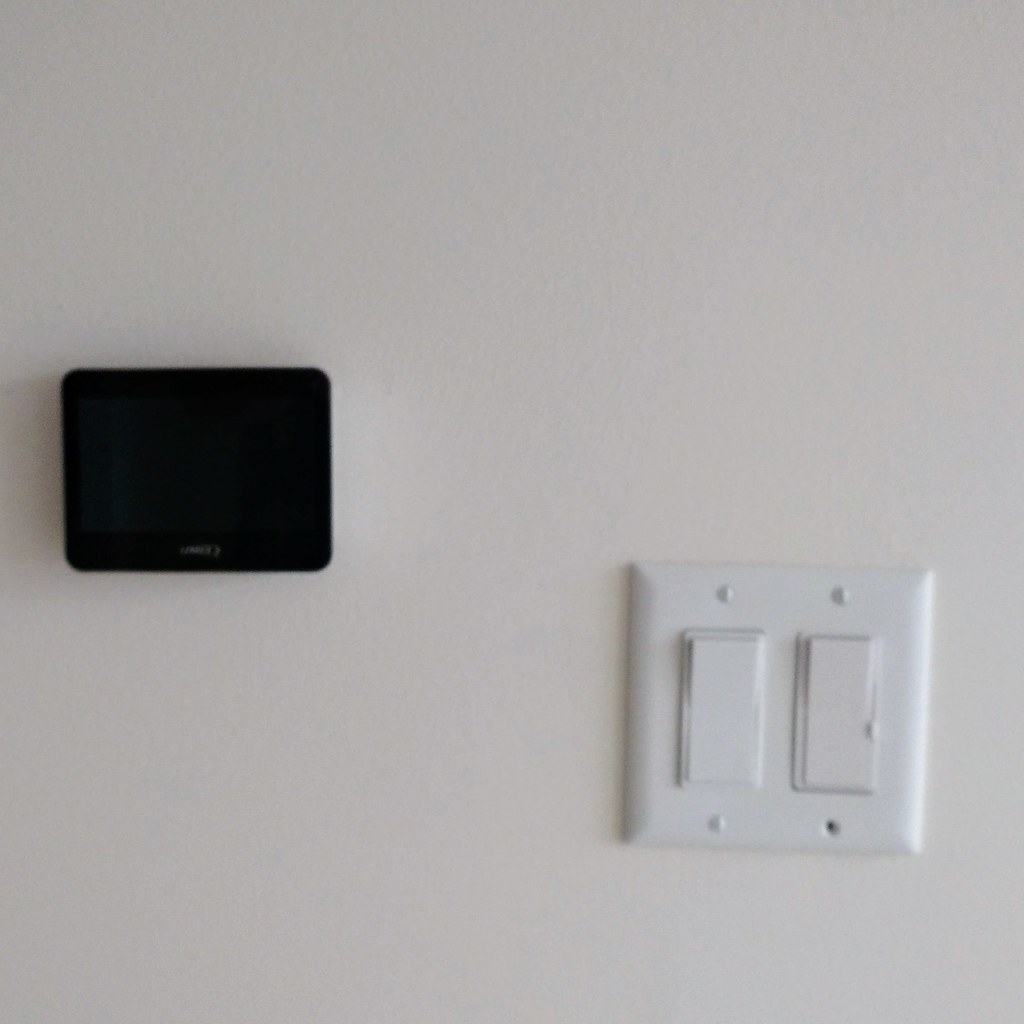The image features a white wall with a basic light switch and a small black box positioned above it. The light switch comprises two buttons, one for turning the light on and one for turning it off. It is held in place by four screws, although the bottom right screw is missing, leaving an empty hole. The wall itself is plain white, providing a stark contrast to the switch and the black box above.

The black box has some illegible lettering beneath it and appears quite simple in design. It may serve as a small pad for an alarm system, but its exact purpose is unclear. The overall color scheme of the image is monochromatic, featuring only white and black. Besides the light switch and the black box, there are no other elements present in the image, making it a minimalist and straightforward composition.